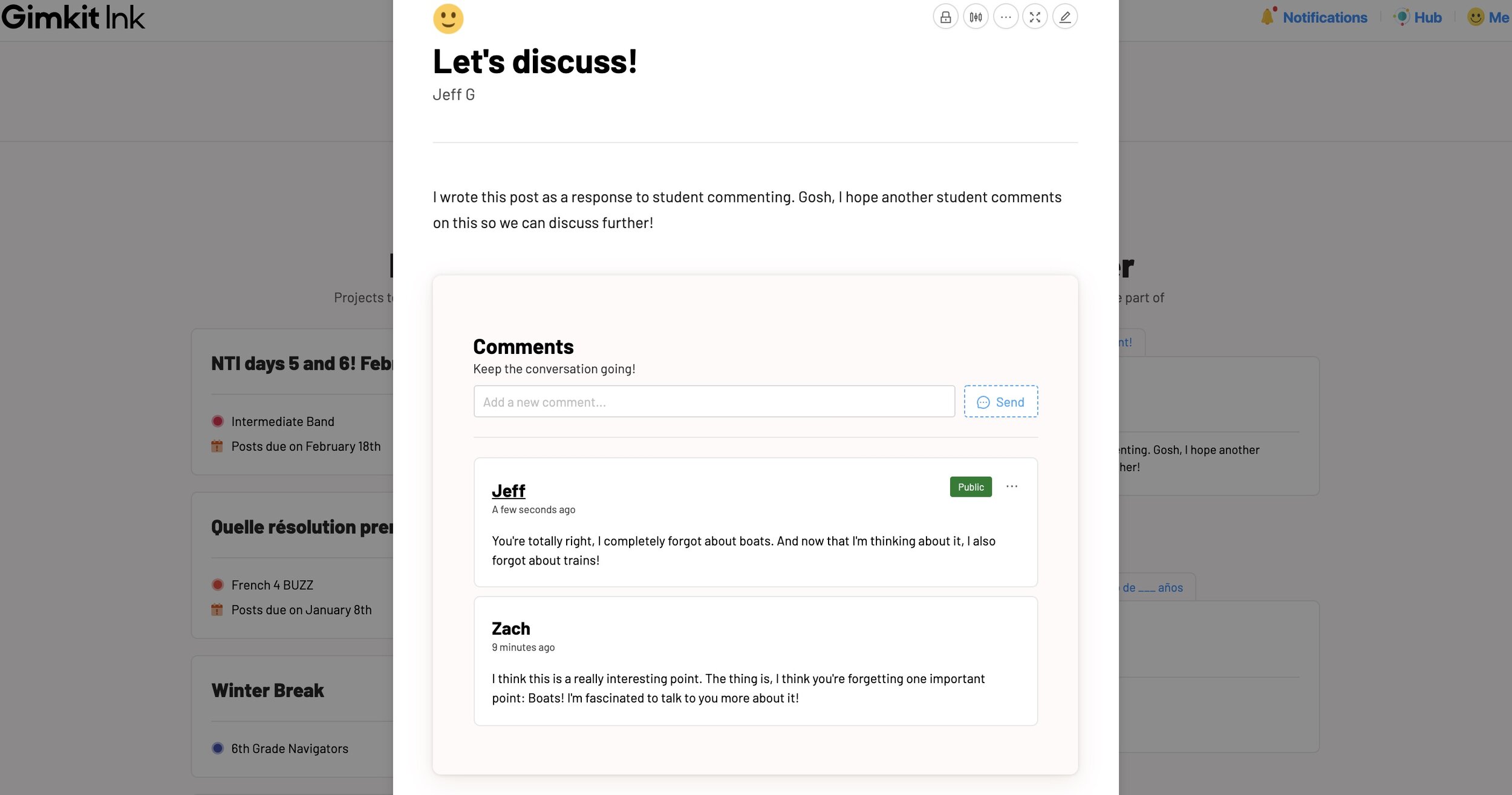### Detailed Caption for the Image

The image displays two overlapping rectangular pictures. The larger, bottom image is a wide rectangle with a gray overlay, and it features "GimKit Inc." written in the upper left corner. Overlaying the larger image is a smaller rectangle positioned in the center, with a white background.

The bottom image appears to be a digital notice, partially obscured by the smaller rectangle. Visible texts include "NTI Days 5 & 6 Intermediate Band," with posts due on February 18th, and "French for Buzz posts due on January 8th." The heading "Winter Break" is also visible, followed by "8th Grade Navigators."

The smaller, overlaid rectangle contains a discussion interface. In the upper left corner is a yellow smiley face icon next to the prompt "let's discuss." Below this prompt is the name "Jeff G," followed by the text: "I wrote this post as a response to student commenting. Gosh, I hope another student comments on this so we can discuss further." Underneath, there is a call to action: "Keep the conversation going," along with a text box labeled "add a new comment."

Further down, there are sample comments, starting with "Jeff" who posted "a few seconds ago," stating: "You're totally right. I completely forgot about bolts, and now that I'm thinking about it, I also totally forgot about trains." Below this, "Zach" commented nine minutes ago: "I think this is a really interesting point. The thing is, I think you're forgetting one important point. Bolts. I'm fascinated to talk to you more about it."

This detailed arrangement and contents suggest an educational platform or discussion forum where students and educators can interact and engage in topic-based conversations.